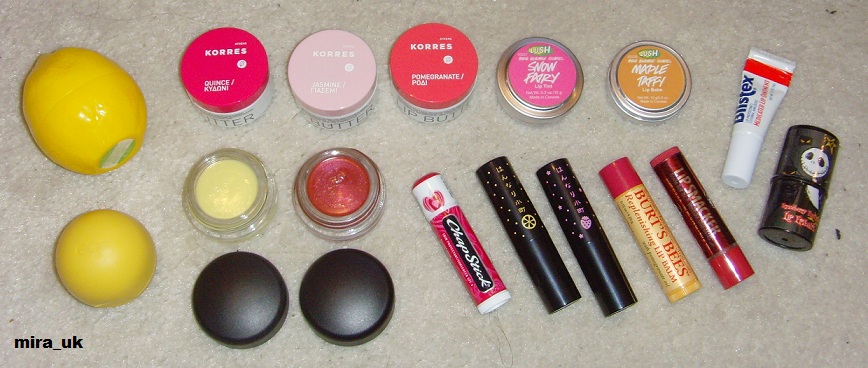The picture showcases an array of approximately 15 different lip glosses and balms, among other beauty products, laid out on a light gray carpet. Prominently featured are a variety of brands and types such as pots, sticks, and open containers. The pots, including those from Lush and Kores, come in colors like a purple-y pink and orange. The sticks include a red and black Chapstick and a yellow and red Burt's Bees. A unique lemon-shaped product catches the eye on the left side, shiny and yellow. Several cylindrical containers with colorful lids are also visible, with labels like "K-O-R-R-E-S," "Snow Fairy," and "Maple Fairy." Noteworthy is the text "MIRA_UK" at the bottom left in black, and the presence of other makeup products like Blistex, adding to the diverse collection. Additionally, a Jack Skellington-themed item appears on the right, contributing to the eclectic assortment of beauty essentials.